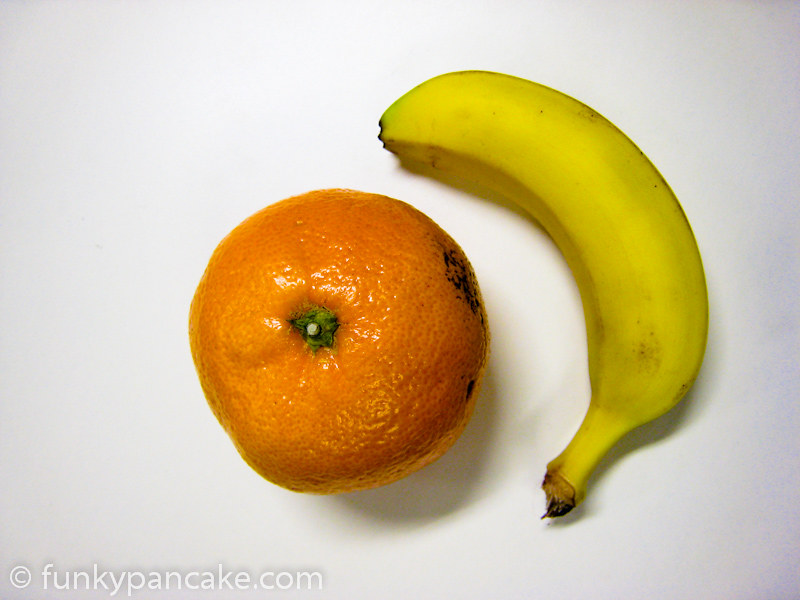**Description:**

This photograph features a meticulously arranged still life of fruit set against a pristine white background. The backdrop gradient transitions from a soft silver at the corners to a subtle gray, ultimately merging into a bright white at the center, which strikingly enhances the vivid colors of the fruit. 

Central to the composition is a plump orange, gleaming under the subtle lighting which also casts a delicate reflection. The orange is topped with a green stem area, although there is a small black blemish on its side that suggests it may be overripe. 

Adjacent to the orange, positioned at approximately the three o'clock mark relative to it, is a short, stubby banana. The banana's predominantly yellow peel is accented with a touch of green at its base and several scattered brown spots, indicating varying stages of ripeness.

The seamless arrangement of the orange and banana suggests a form-fitting alignment, enhancing the visual harmony of the composition. 

At the bottom of the image, a discreet watermark and copyright notice in white text reads "© funkypancake.com," indicating the source or creator of the photograph.